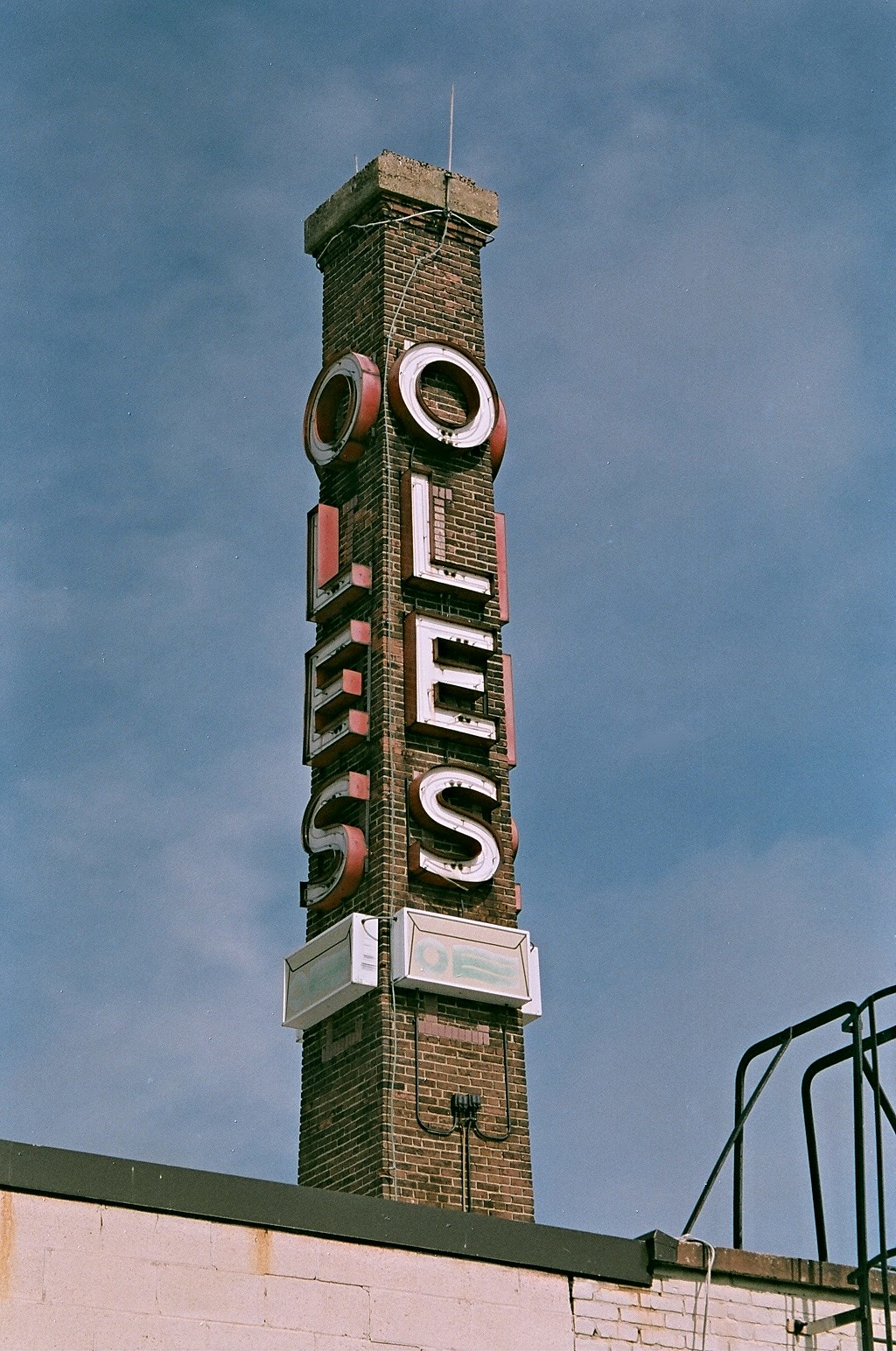The photograph captures a detailed daytime view of a weathered, brick chimney stack, which likely dates back many years, suggesting an old factory building. The chimney, constructed from brown brick, stands on a flat roof, protruding prominently above the structure. On one of its faces, the neon letters "O-L-E-S" are vertically arranged, with a box-shaped element beneath the "S." This neon signage likely illuminates at night, making the name visible from multiple angles. Two slender white antennas extend from the chimney's top, and several wires are connected to its structure. On the right side of the photo, there is a steel structure resembling an emergency fire escape ladder, accentuating the industrial feel of the scene. The background features a partly cloudy blue sky, adding depth to the overall composition. The orientation of the photo is portrait, emphasizing the height of the chimney stack, which appears about four to five times taller than its width.